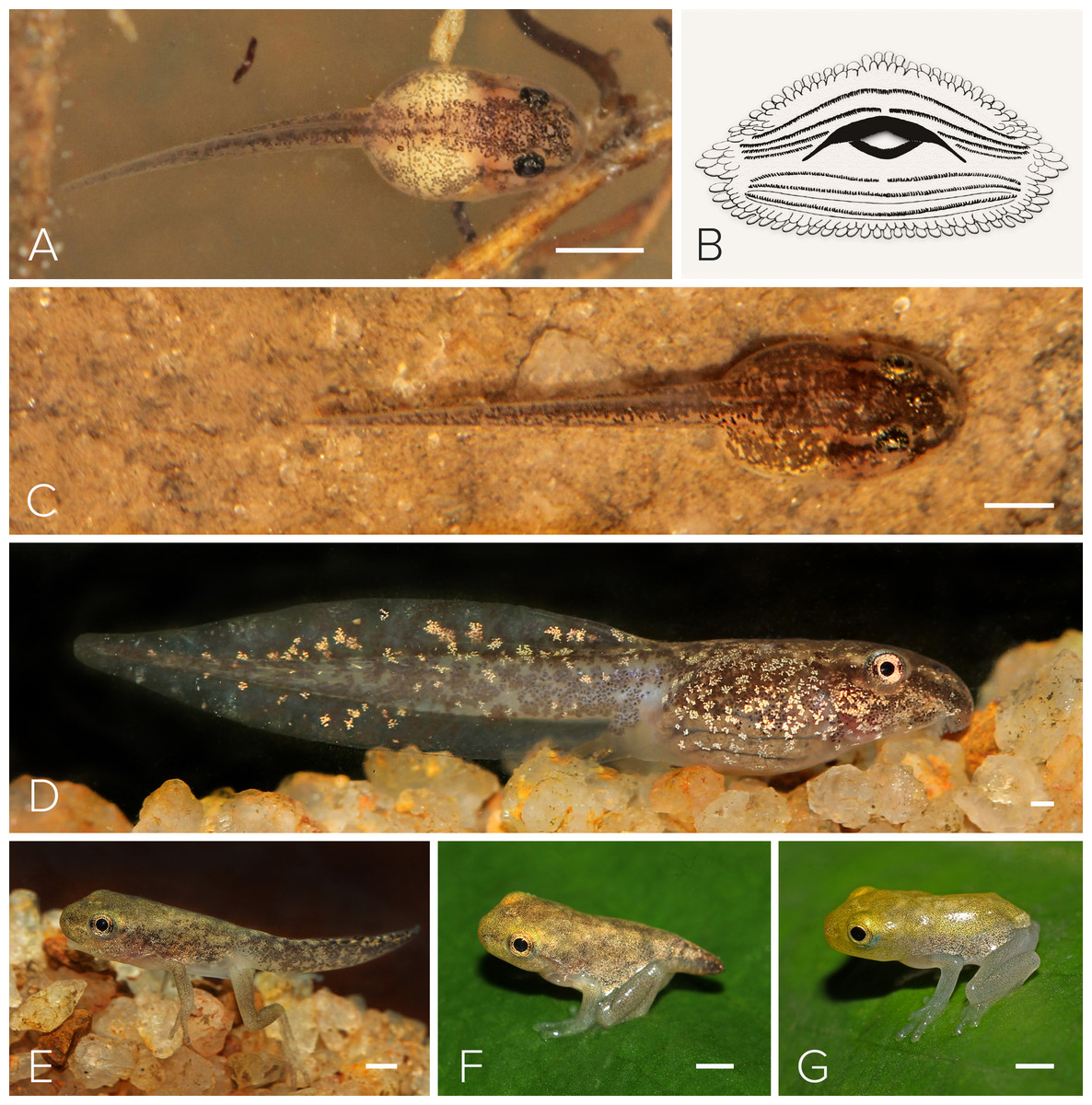This is an elaborate illustration depicting the early stages of the life cycle of a tadpole transforming into a frog. The series includes seven images, each marked with a letter from A to G, showcasing the gradual metamorphosis. 

In the first image labeled A, a small tadpole is seen swimming in pond water, possibly feeding on detritus. This is the initial stage, characterized by its short tail and round, simple body. 

Image B shows the tadpole slightly larger, still in black and white, indicating its early growth phase. 

By image C, the tadpole is more developed with a longer tail and distinct black eyes, positioned at the bottom of its aquatic environment, surrounded by sand or small pebbles.

In image D, the tadpole’s tail appears thicker as it continues to grow, still interacting with a sandy or rocky bottom.

Image E marks a significant transformation, where the tadpole begins to sprout legs, starting to resemble a young frog. This stage illustrates the tadpole on differently colored pebbles as its body structure starts transitioning.

In image F, the transformation advances further; the creature looks more like a frog with budding legs, showing only a small remnant of its tail as it rests on a green leaf.

Finally, image G presents the fully developed frog, now with no tail, and an iridescent yellowish-clear coloration with black eyes. At this stage, the frog is fully formed, completing its incredible journey from a tiny tadpole to a fully recognizable frog.